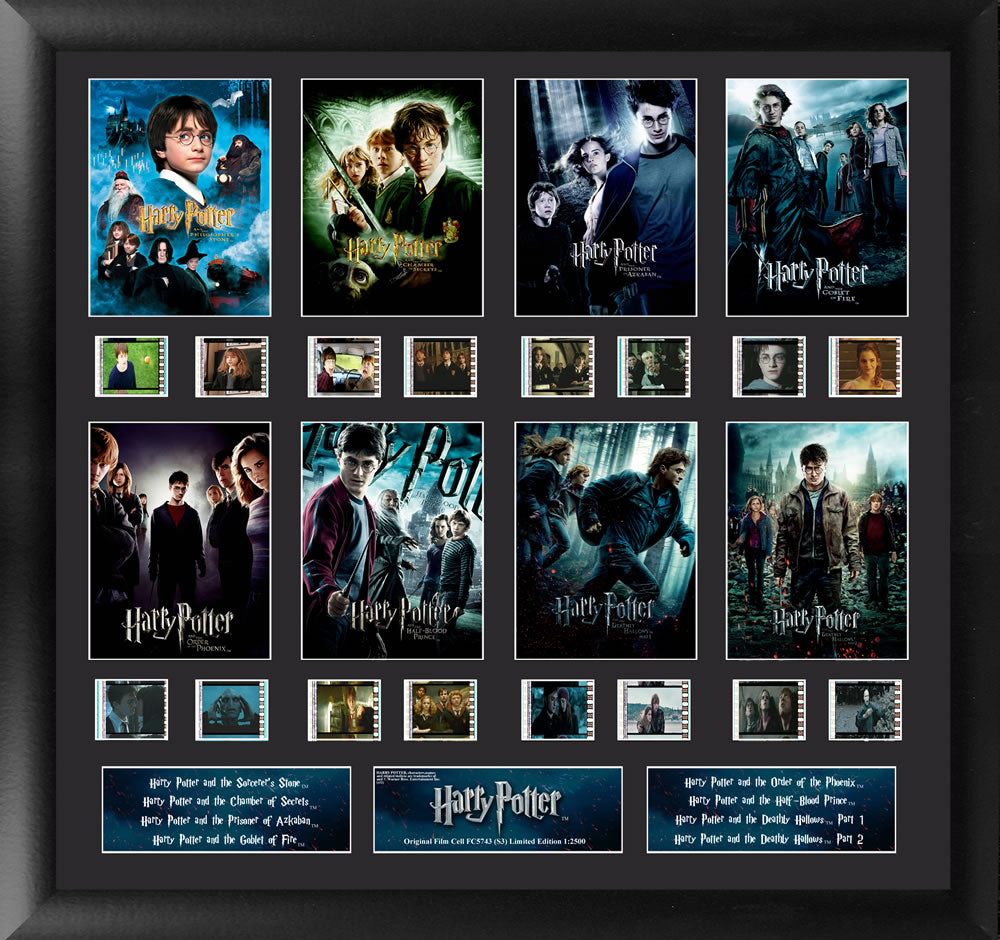The image depicts a framed Harry Potter collectible item, meticulously designed for display on a wall. The black frame encloses a gray background, which enhances the vibrant colors of the contents. Arranged in a grid layout, eight postcard-sized movie posters represent each of the Harry Potter films, organized left to right in two rows of four. Beneath each poster are two inset snippets of film reel stills, appearing as miniature frames that capture specific moments from the movies, totaling 16 film snippets. At the bottom of the frame, three text boxes provide additional details: the central box displays the iconic "Harry Potter" title, while the left and right boxes list the titles of all eight movies, from "Harry Potter and the Sorcerer's Stone" to "Harry Potter and the Deathly Hallows Part 2." This item, likely cherished by fans and collectors, brings together all the Harry Potter films in a visually striking, commemorative display.